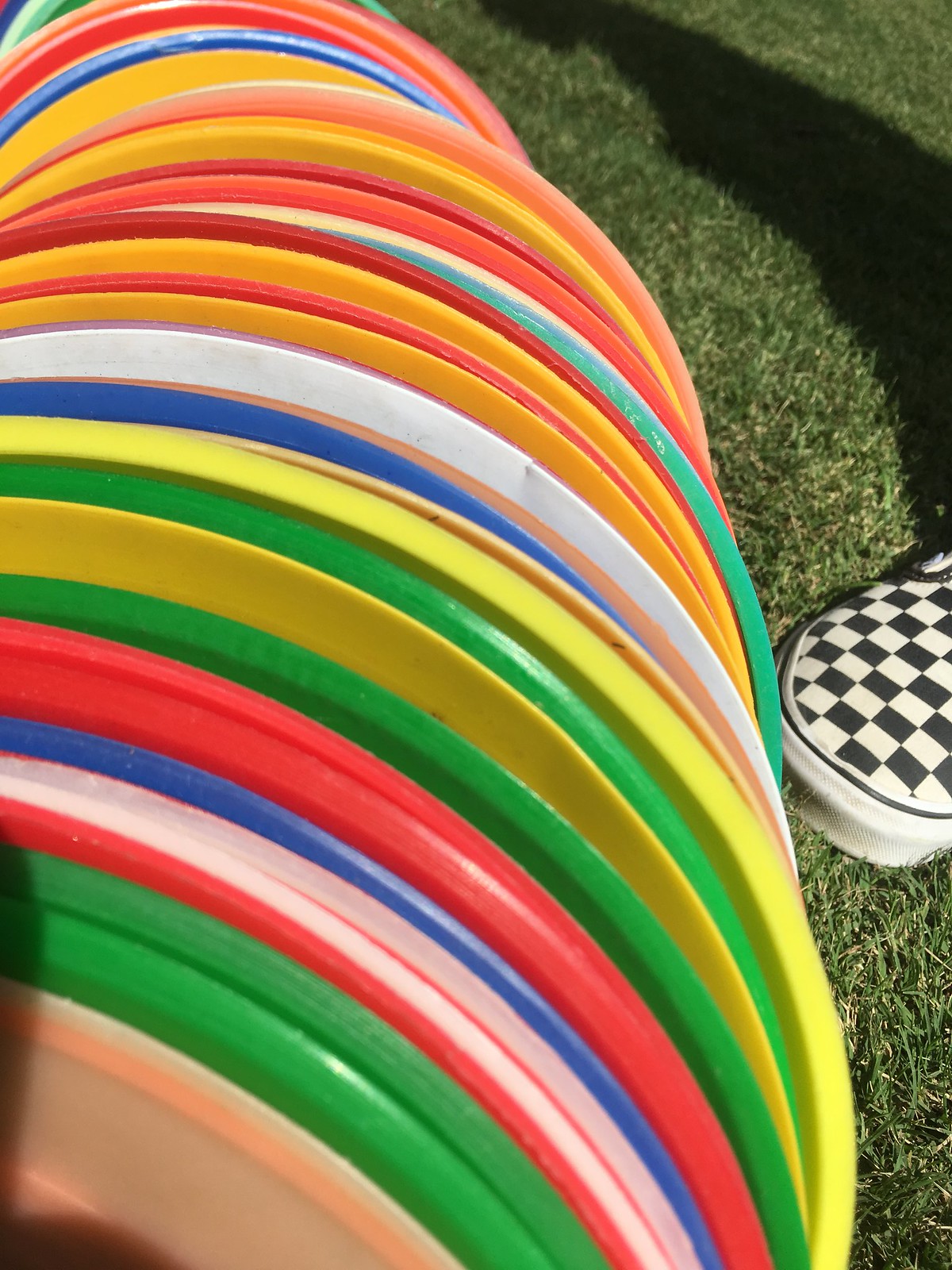This outdoor photograph showcases a vivid scene predominantly filled with an array of colorful frisbees standing on their edges. These frisbees are not perfectly aligned, creating a dynamic pattern across the left and center of the image. They feature a spectrum of hues including pink, green, red, blue, yellow, white, orange, turquoise, maroon, and purple. On the right side, green grass is visible, along with the shadow of an individual. The sneaker belonging to this person is partially visible; it is a slide-in tennis shoe with a black and white checkerboard pattern. The overall atmosphere suggests a bright, sunny day.